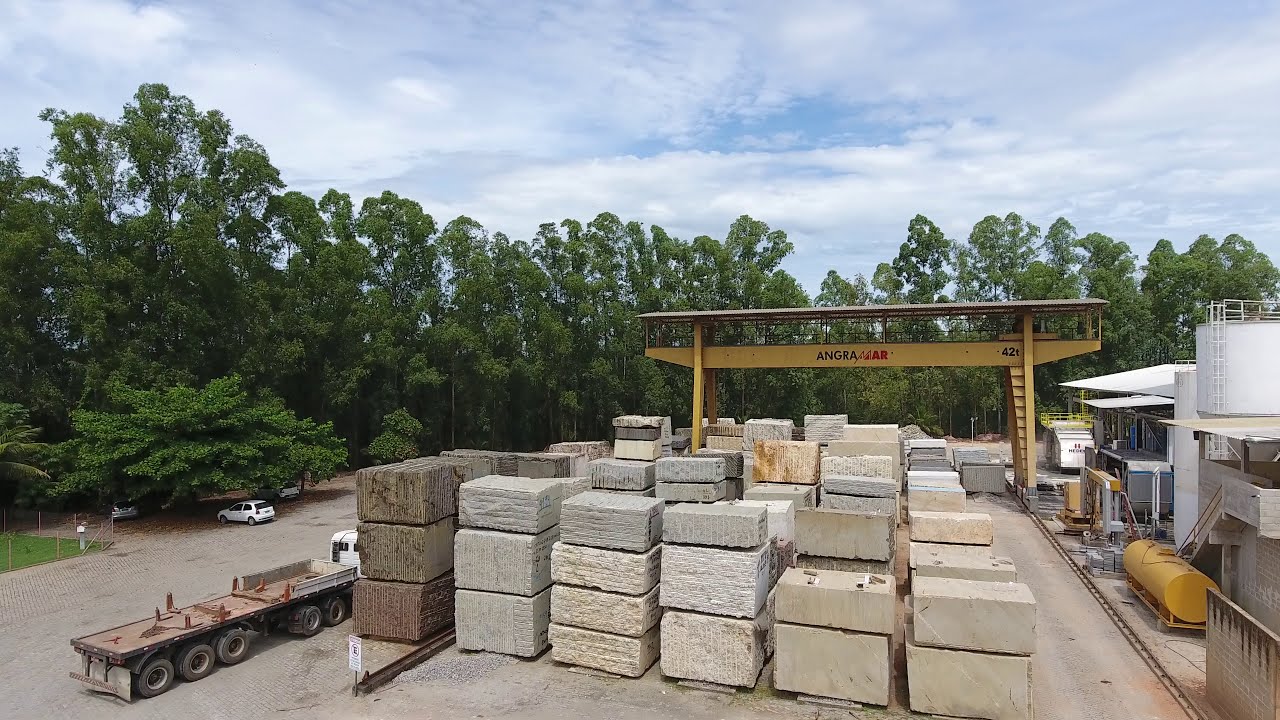This detailed exterior color photograph captures a cargo or construction yard on a bright sunny day with a blue sky dotted by thin white clouds. The expansive ground in the foreground is dominated by neatly stacked large stones of varying shades—gray, dark brown, and cream—arranged in rows that stretch across the yard. The stones, about as tall as a truck, have a striated texture, indicating compressed material or carved lines.

On the right side of the image, there are cylindrical industrial buildings, including a prominent yellow cylindrical tank likely used for gas storage. Nearby, there is a metal rampway emblazoned with the black letters "ANGRA" and additional red letters beyond it. A large white truck with a long flatbed trailer, featuring at least six pairs of wheels, is stationed to the left, alongside a white car.

Tall, green trees border the area, enhancing the natural backdrop. The scene is bathed in sunlight, with the sky above featuring patches of blue interspersed with white clouds, none of which obstruct the sun, adding a bright and clear atmosphere to the photograph.